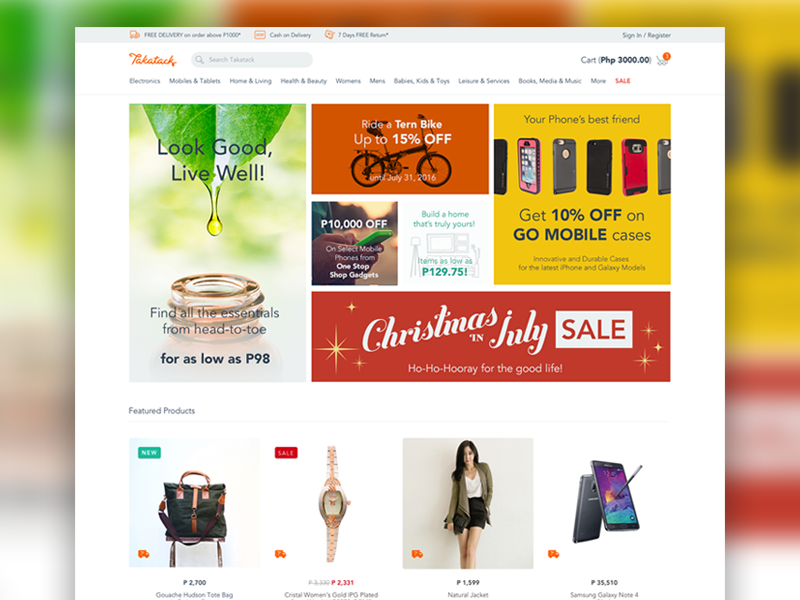The image features a layered composition. The background presents a blurred, colorful scene that seems to resemble the aisle of a department store, painted with bright hues of yellow, red, and green. Superimposed on this background is what appears to be a screenshot from a website called "Takattack" (spelled T-A-K-A-T-A-C-K), identifiable by its orange text logo in the upper left corner.

The website UI showcases a top search function and several clickable links that categorize various shopping sections, including "Home and Living," "Mobile and Tablets," "Electronics," "Health and Beauty," "Women's," and "Men's" products. Below these categories, the website display continues with a grid of images arranged in square and rectangular formats, collectively forming a long rectangular banner.

One notable section of this banner reads "Live good, live well," advertising a range of essentials starting at P-98, accompanied by an image of a leaf dropping oil into a bottle. Another prominent banner stands out with "Christmas in July Sale," presented in striking red with white text.